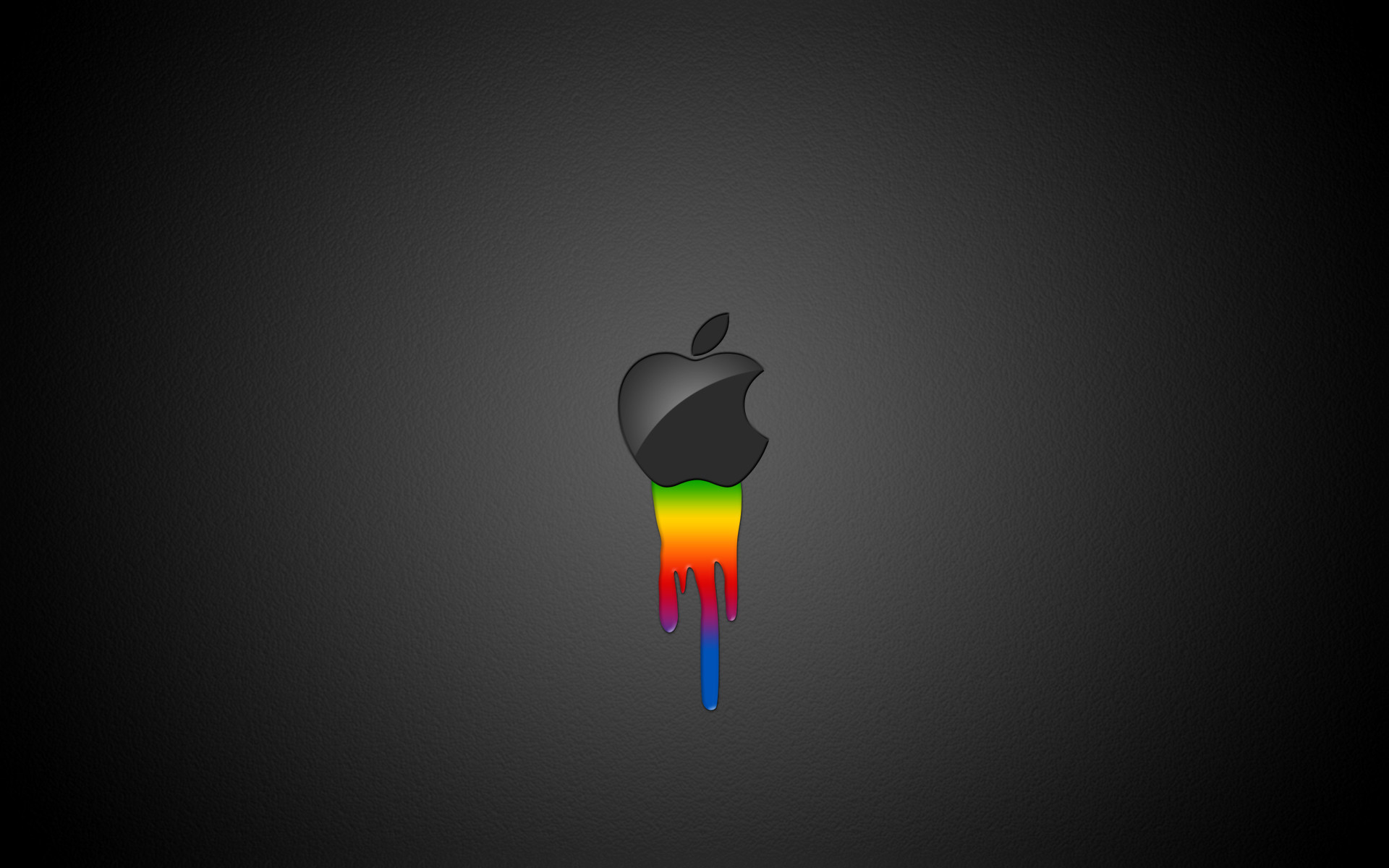In the image, there is a predominantly black background that fades to gray towards the center, which creates a subtle spotlight effect highlighting the main subject. At the very center of the image, there is a stylized Apple logo, reminiscent of the iconic branding by Apple Inc. The Apple logo itself is black with a lighter gray shading on the upper portion and a distinct leaf at the top. Notably, the logo features a semi-circular bite mark on its right side. Emanating from the base of the logo is a series of rainbow-colored paint drips, cascading downward in a vivid spectrum of green, yellow, orange, red, purple, and blue. These colorful drips create an uneven, streaked pattern beneath the logo, giving the illusion of liquid paint leaking from the bitten apple. The overall texture of the image suggests it could be a close-up of a MacBook's surface, with the focus solely on the dynamic interplay between the stark monochrome logo and the vibrant, multi-colored paint drips. The edges of the image are enveloped in deep black, further emphasizing the central Apple logo and its striking, flowing colors.